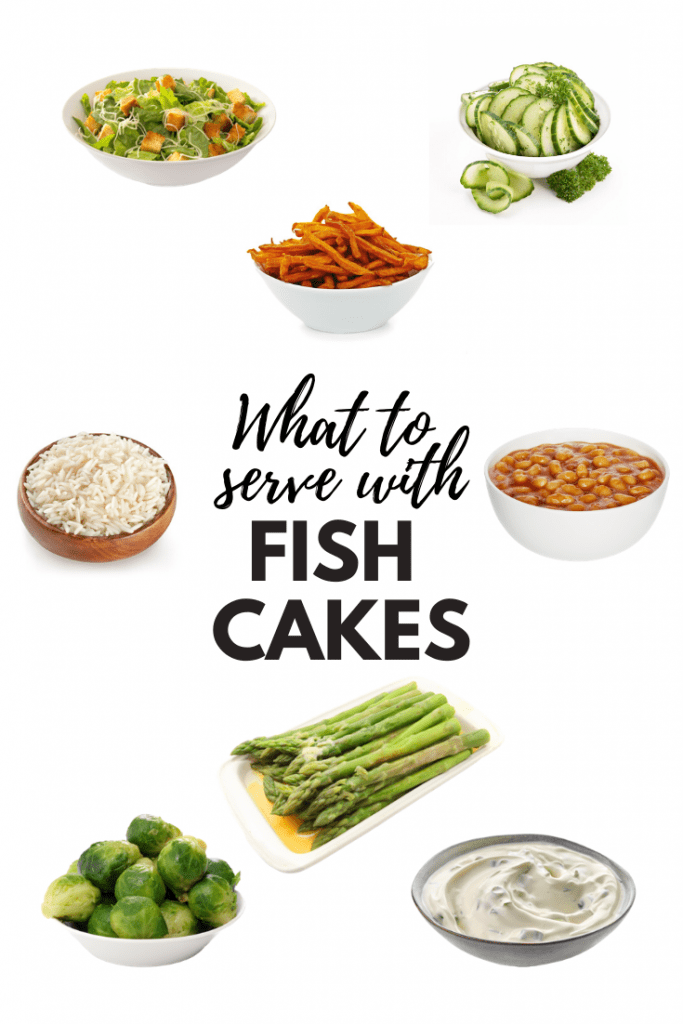This image, possibly an advertisement or flyer, features a central theme on a white background with black text. The text, set in a computer-like recursive handwriting, reads "what to serve with" and beneath it, in bold, uppercase Arial font, "fish cakes." Surrounding this central text are various suggested side dishes arranged in a cohesive layout.

- In the top left corner, a white bowl contains a Caesar salad adorned with croutons and grated Parmesan cheese.
- The top right corner showcases a bowl of intricately spiral-cut cucumbers, resembling a cucumber salad.
- Centrally located just below these two dishes is a bowl filled with orange sweet potato fries.
- To the left of the main text, a small bamboo or wooden bowl holds a serving of white rice.
- On the right side, there’s a white bowl filled with baked beans.
- Directly below the text in the center is a white plate of asparagus dressed in a buttery sauce.
- The bottom left corner presents a white bowl of Brussels sprouts.
- In the bottom right corner, a grey or metallic bowl holds a creamy white sauce, likely tartar or ranch dip.

All these elements are meticulously organized around the central question of what to serve with fish cakes, providing a visually appealing and comprehensive guide to complementary dishes.